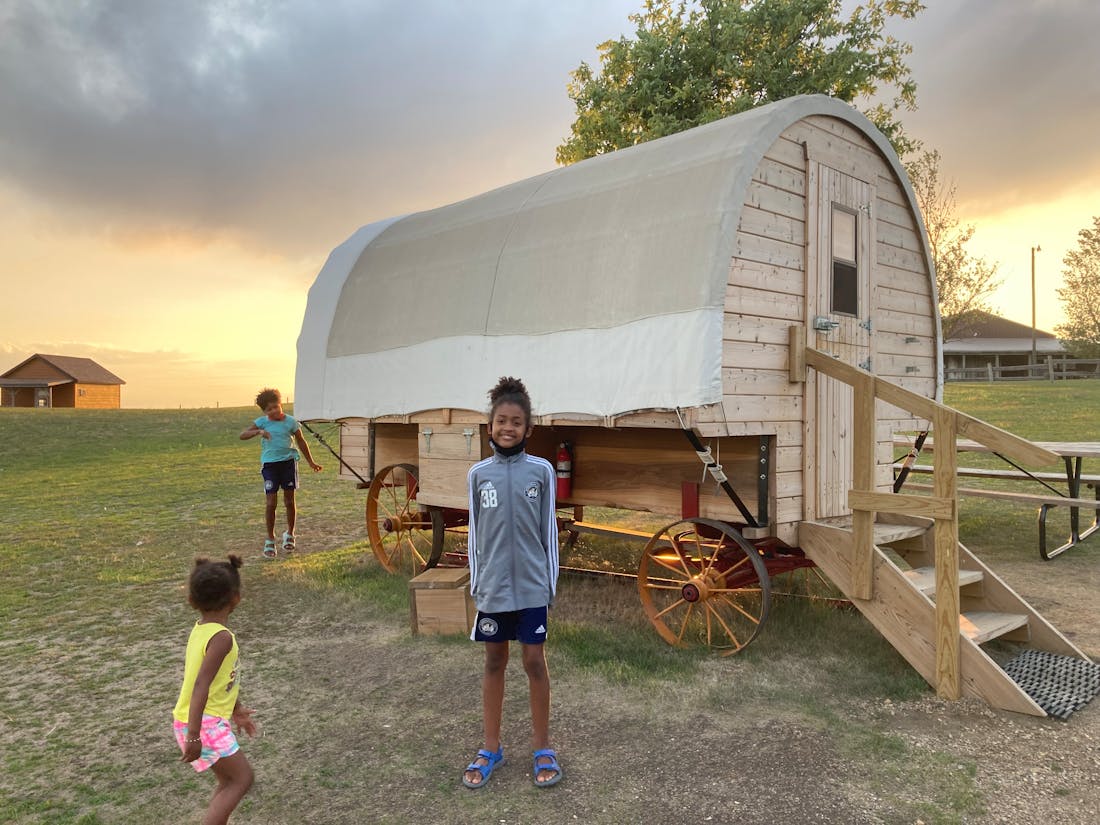Three children are central in the photo, all directing their gazes towards the viewer. The youngest is a small girl with a dark complexion, wearing a yellow shirt and pink and white shorts. She looks back towards an older child, who wears a cyan shirt and blue shorts. The third child, smiling brightly, is dressed in a gray sweatshirt, blue shorts, and blue Crocs sandals. Behind them is a wooden wagon with brass wheels, now converted into a small room with a white tarp cover and a door accessible by three steps. The wagon resembles a covered wagon from the past, repurposed into a tiny rolling home, which could be an imaginative play area for the children. The scene appears to take place on a grassy area, possibly a ranch, evidenced by a log home in the far distance, a picnic bench nearby, and a solitary tree's top visible behind the wagon. A fire extinguisher is attached to the side of the wagon, and a vast gray cloud spans the sky with pale yellow sunlight in the background.